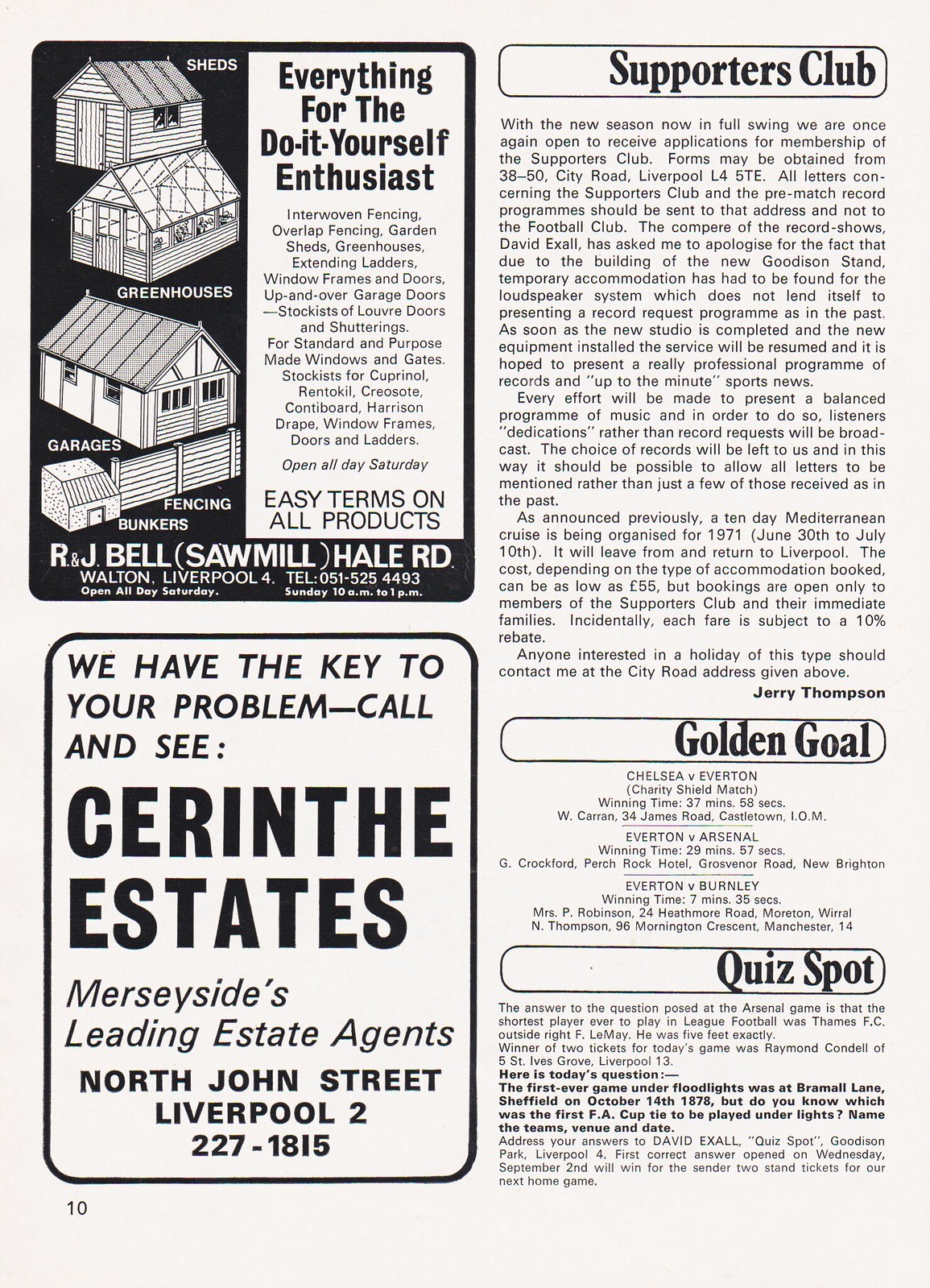This image captures a page from an old magazine or newspaper, featuring both advertisements and editorial content. On the left side, two prominent advertisements stand out. The first ad is for R. & J. Bell Sawmill, located on Hale Road, Walton, Liverpool, offering a range of products for the do-it-yourself enthusiast. It lists items such as sheds, greenhouses, garages, fencing, and bunkers, and highlights easy payment terms on all products. The ad proclaims, "Everything for the Do-It-Yourself Enthusiast," and enumerates their offerings, including interwoven fencing, overlap fencing, garden sheds, greenhouses, extending ladders, window frames, and doors. Below this, another ad declares, "We have the key to your problem," urging readers to visit Serente Estates, Merseyside's leading estate agents, located at North John Street, Liverpool 2, with the contact number 227-1815.

On the right side, the editorial content is divided into several sections. The top section is titled "Supporters Club" and comprises four paragraphs of text attributed to Jerry Thompson, although the text itself is too small to read. Following this, the "Golden Goal" section likely details sports scores, including a mention of Chelsea vs Everton, spread across three paragraphs of similarly minuscule text. The final section, titled "Quiz Spot," includes two more paragraphs of small, illegible text. This page is identified as page 10 of the publication.